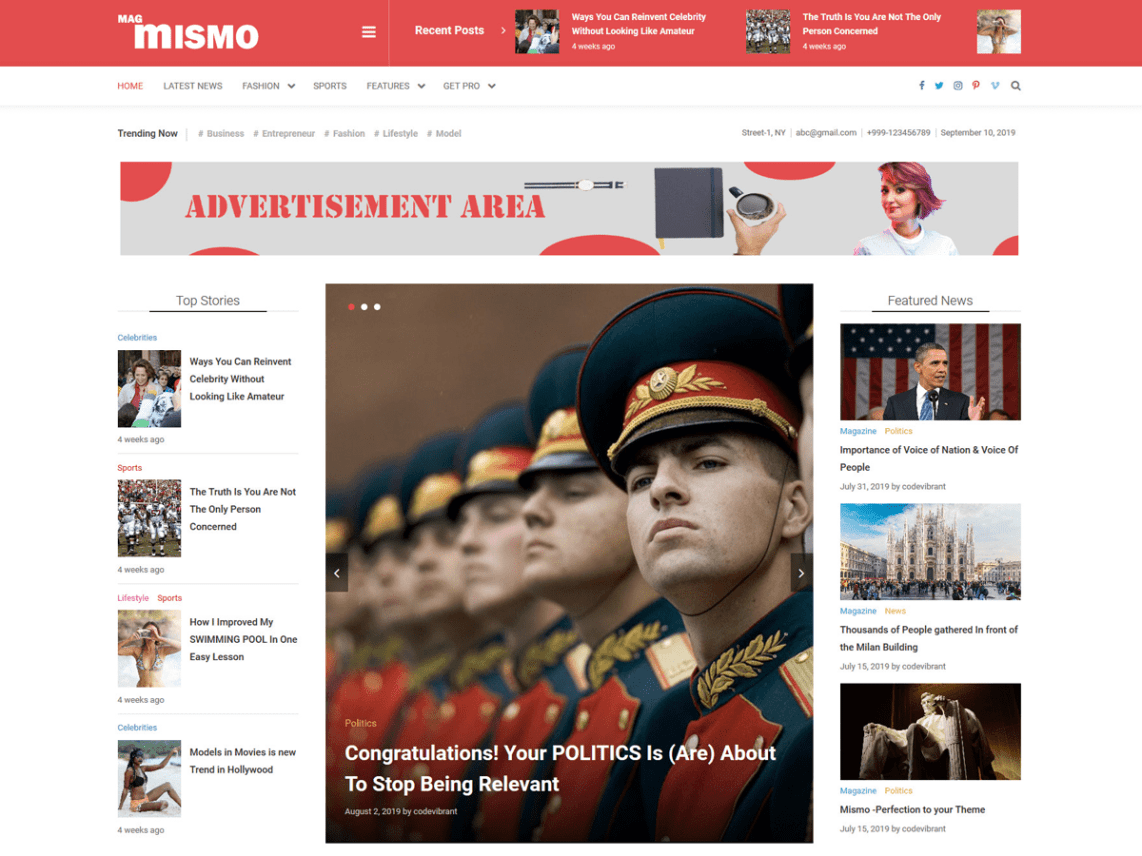The webpage for MAG-MISMO is presented with a user-friendly and visually engaging layout. At the top of the page, clickable features are prominently displayed, allowing easy access to various sections. Featured elements include recent posts accompanied by vibrant photos and engaging titles, as well as a section dedicated to celebrity retirement, although part of the text is blurred and unreadable.

Just below an orange banner, there are several clickable choices including Home, Latest News, Fashion, Sports, Features, and Get Pro. Beneath this banner, there's a 'Trending Now' section showcasing categories such as Business, Entrepreneur, Fashion, Lifestyle, and Model.

On the right side of the same banner line, additional options are displayed including phone numbers, the date (September 16th, 2019), and information about the current volume of the publication. Following this, a light gray border designates an advertisement area, featuring an image of someone holding a cup of coffee and a red-haired girl wearing a white t-shirt.

Several story options are displayed with corresponding photos, though some content is blurred and difficult to read. In the central part of the page, a larger image features members of an army dressed in red, blue, beige, and gold uniforms with hats and caps. The headline associated with this image reads, "Congratulations, your politics is (are) about to stop being relevant."

To the far right, there are three other featured stories. The first highlights "Importance of the Voice of the Nation and Voice of the People," illustrated with a photo of Barack Obama. The second story caption reads, "Thousands of people gathered in front of the Milan building," accompanied by an image of buildings. The final story features a statue resembling Abraham Lincoln, with the title reading, "Mismo, perfection to your theme."